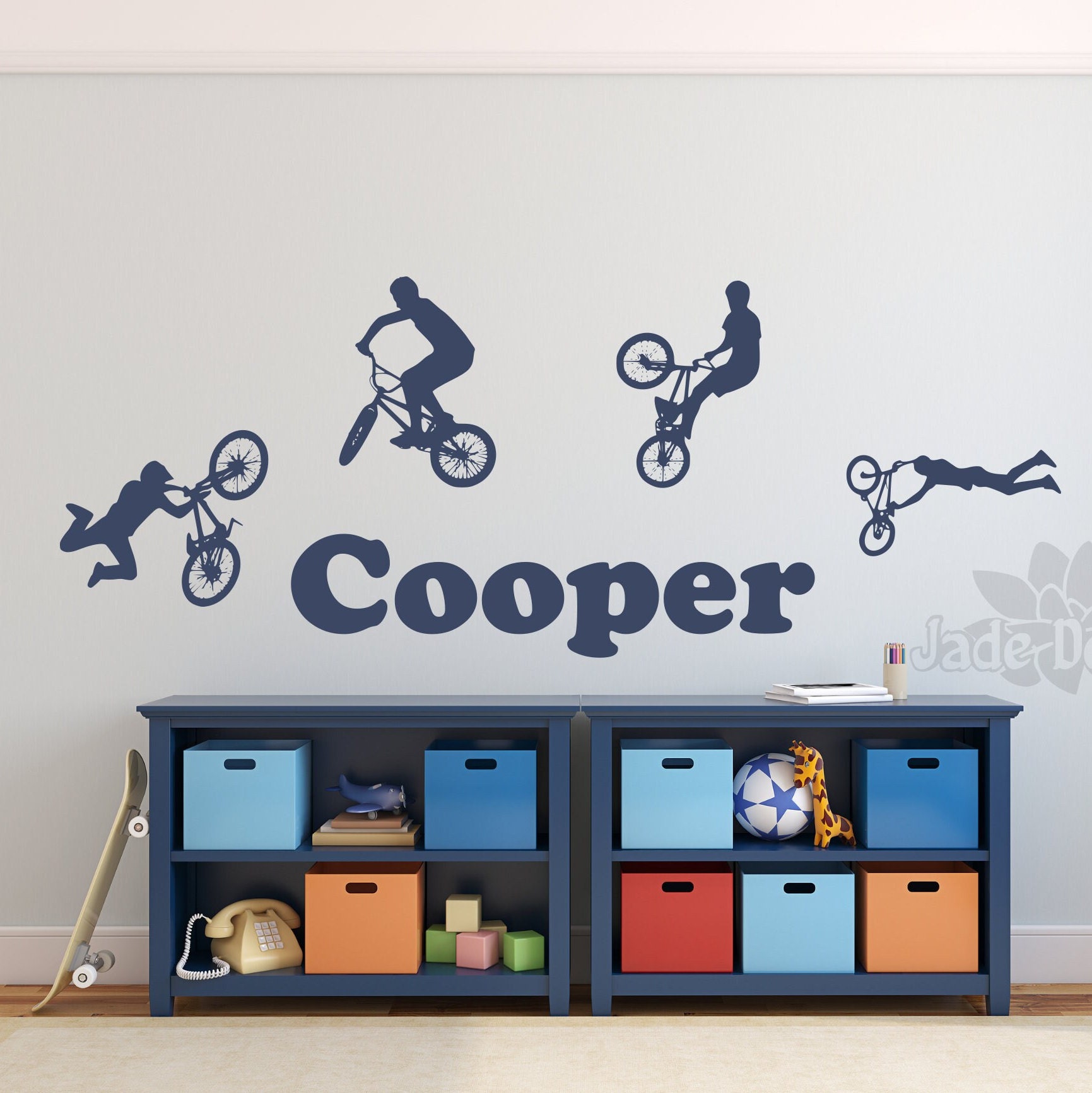The image depicts a neatly organized child's room with a professional, symmetrical layout accentuated by artistic touches. Central to this setup are two identical blue storage shelves with built-in cloth drawers. Items such as a plastic phone, airplane, blocks, a soccer ball, a toy giraffe, and a cup with colored pencils adorn the shelves, while a pair of books rests on top of the right shelf. A white skateboard leans against the left side of the storage units.

The background features a white wall embellished with a stenciled mural showcasing four silhouettes of a figure performing BMX bike tricks, sequentially arranged. Above the shelves, in bold, dark blue stenciled letters, is the name "Cooper," suggesting the room belongs to a child named Cooper. The entire scene is set on a polished wooden floor, contributing to the overall crisp and tidy appearance of the room.